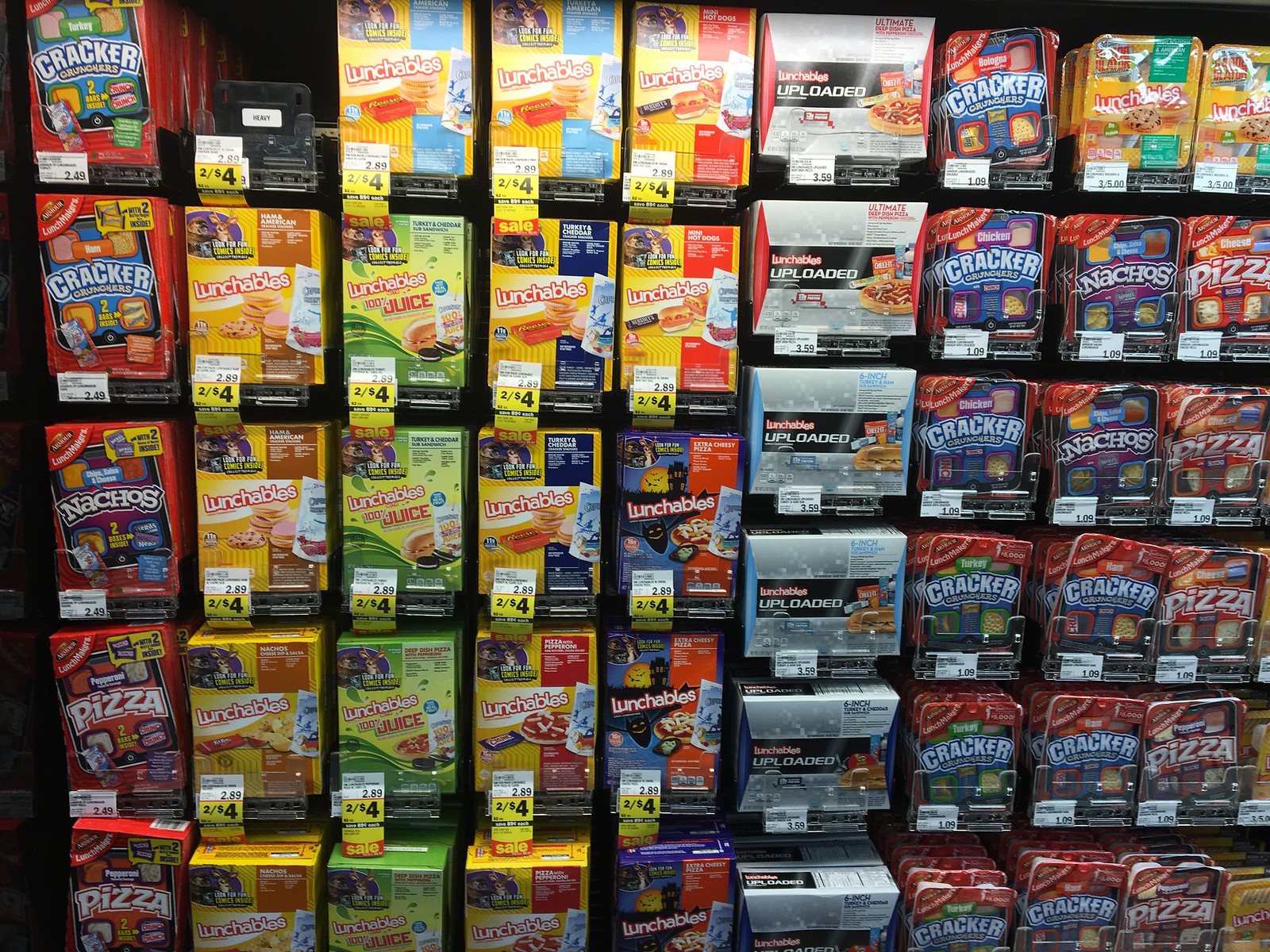This photograph showcases a well-stocked section of a grocery store dedicated to portable lunch options. Dominating the scene are nine neatly arranged columns of various brands and types of ready-to-eat meals, with the partial appearance of a tenth column. In the foreground, the display begins with an assortment of cracker-based lunch kits featuring nachos and pizza. Adjacent to these, a significant portion of the display—about four columns—is filled with a diverse variety of Lunchables, offering combinations of turkey and ham sandwiches, crackers, chips, and desserts. As the display progresses, other competing brands of lunch kits make their appearance, providing similar options. Notably, in the center, there's a larger box labeled "Lunchables Uploaded," signifying an even more substantial portable lunch kit. The vibrant packaging and variety of options emphasize convenience and variety for quick and easy meals on the go.